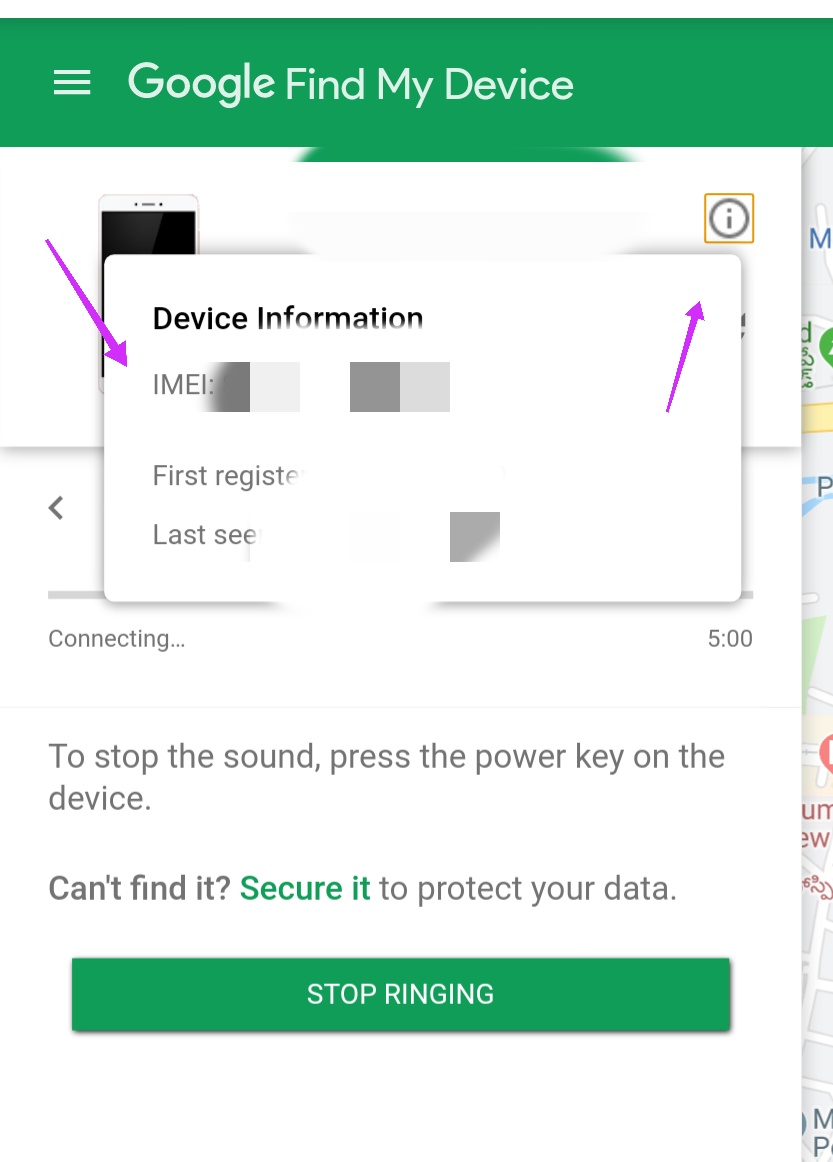A pop-up window labeled "Google Find My Device" appears overlaying another webpage that features a map. The pop-up, which aims to help users locate their lost devices, displays various sections of information in gray and dark gray bars. At the top, there is a gold box with a gray circle featuring an eye icon, indicating surveillance or tracking. The interface shows device details with labels such as "First Registered" and "Last Seen." 

There are two arrows within the interface: one pointing up towards the gold box and another indicating connectivity, presumably from a cell phone, stating "Connecting, 5 o’clock." Additional instructions inform users that they can stop the device's sound by pressing the power key. For those unable to locate their phone, directions to secure the device to protect data are provided. A green bar at the bottom of the screen allows users to stop the ringing once the device is found. The overall image is predominantly black and white, with green accents at the top and bottom serving as borders.